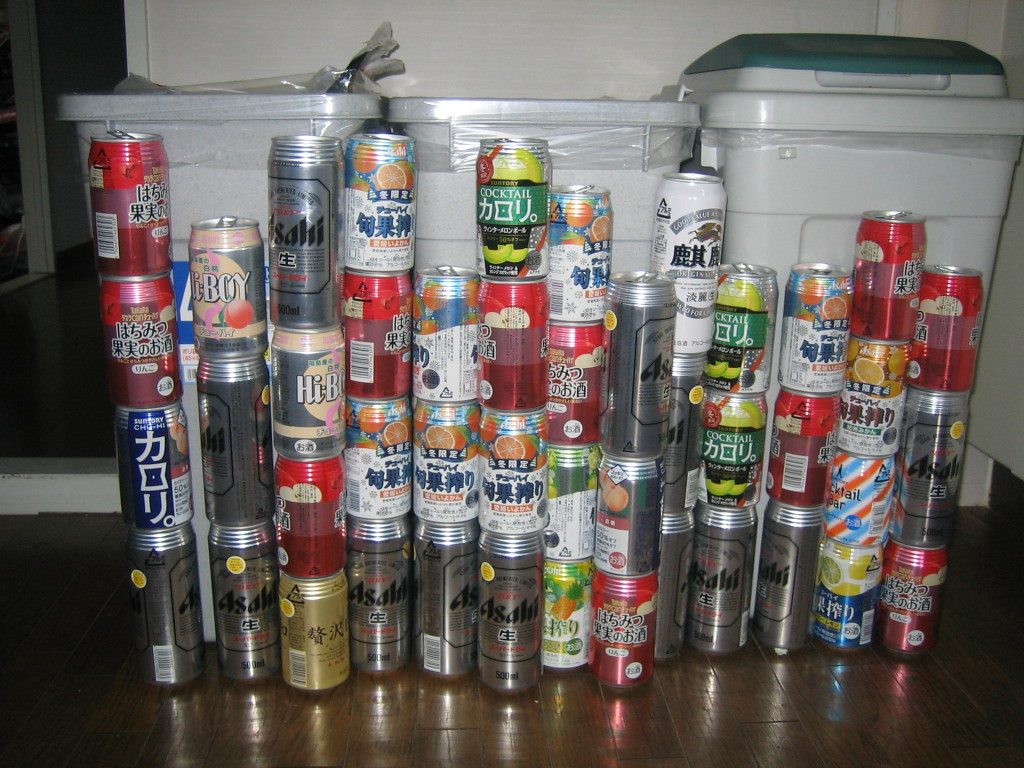The image depicts an orderly arrangement of various colored cans, both single and double-stacked, in front of three white trash cans against a white wall with molding. Each trash can contains a clear plastic bag; the first two are lidless, while the third features a white lid with a green flip piece for disposing of waste. The cans, likely empty given that some tabs are open, form vertical stacks of three to four cans high and are horizontally lined up. They prominently display labels such as 'Hi Boy' and 'Cocktail,' with much of the writing appearing to be in a foreign, possibly Asian, script. The setup suggests a photo shoot, emphasizing the cleanliness and arrangement on a polished wooden floor. The background also reveals the start of a dark hallway to the left, introducing depth to the scene.